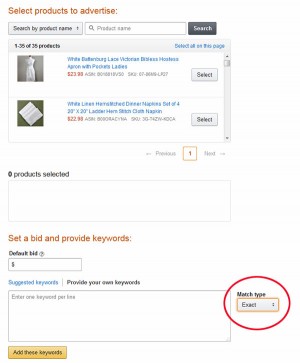The image features a predominantly white background. At the top, a bold red header reads "Select Product to Advertise." Directly beneath this header is a prompt stating "Search by product name," accompanied by a white rectangular input box labeled "Product name" and a dark button with "Search" inscribed in white letters.

Below the search section is a light gray box that displays "1 of 35/35 products" in small, slightly blurry text, with additional blue text to the right of it. Immediately underneath this, the background changes to white, presenting a selection of products.

To the left, there's an image of a dress against a gray backdrop. Adjacent to this image is some blue text detailing the dress and a red price tag. There is also a "Select" button associated with this item.

Further down and to the left, an image of a white object—resembling either a book or pages from a book—is displayed. To the right of this image, similar blue descriptive text is present, along with a corresponding "Select" button.

At the bottom of the image, navigation options are provided, stating "Previous: 1" and "Next: 0" products selected. Additionally, there's an empty text box and a prompt in red that reads "Set a bid and provide keywords," guiding users towards the next steps in their advertising setup.